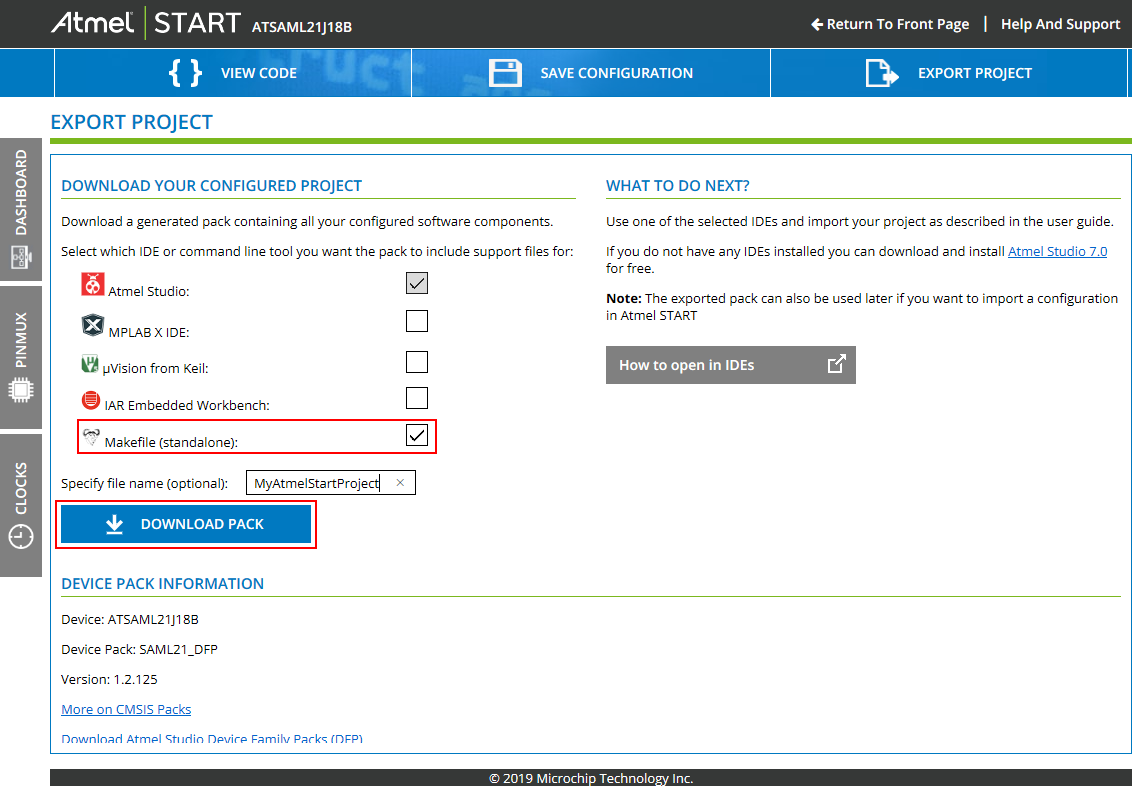The image showcases a software development interface with a prominent black border at the top, labeled "Atmel Start ATSAML21J18B." The header includes navigation options such as "Return to Front Page" and "Help and Support." 

Below this header, there are additional options including "View Code," "Save Configuration," and "Export Project." Centrally located in bold blue capital letters is the "Export Project" button. A green line emphasizes this section, beneath which there is a directive prompting users to "Download Your Configured Project."

Further explained, the interface mentions that users can "Download a generated pack containing all your configured software components." It also instructs users to select their preferred Integrated Development Environment (IDE) or command-line tool to include support files for.

To the right, a helpful guide named "What to Do Next" outlines the necessary steps: users should employ one of the selected IDEs and import the project according to the user guide. For those without a pre-installed IDE, Atmel Studio 7.0 is recommended and available for free download.

Finally, users are advised that "The exported pack can also be used later if you want to import a configuration in Atmel Start." At the bottom of the interface, a gray button labeled "How to Open the IDEs" offers additional guidance.